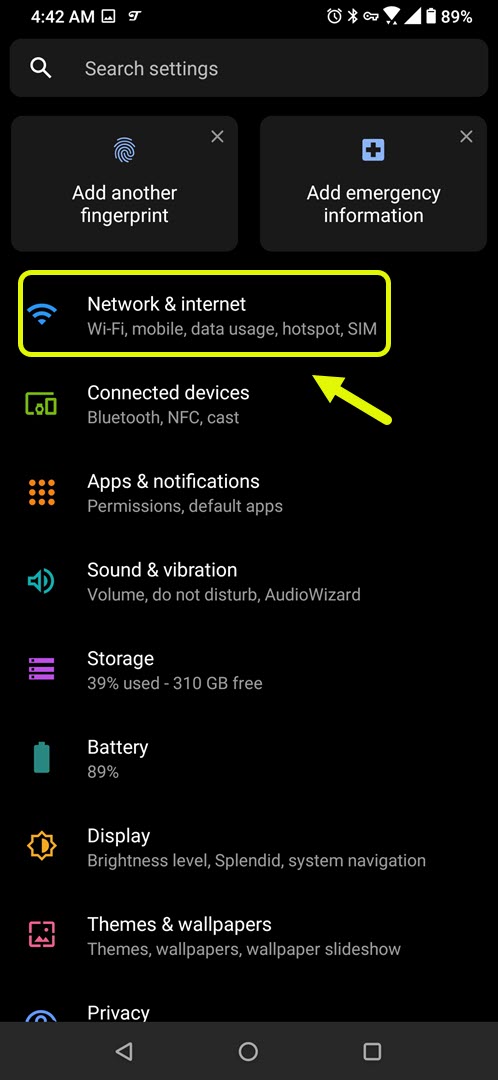Screenshot of a cell phone settings menu

---

This detailed screenshot captures the internal settings menu of a cell phone, evident from the familiar interface elements like the battery icon, battery percentage, and time display in the upper right corner of the screen. The predominantly black background contrasts with the white font, enhancing readability. At the top, right beneath the time display, is a search bar labeled "Search settings."

Immediately below the search bar, there are several quick links. One link allows you to add another fingerprint, indicating that this phone features fingerprint recognition for security. Another link directs users to input emergency information.

Following the quick links is a comprehensive list of settings categories, each offering an array of configurable options:

1. **Network & Internet**: Modify network settings, adjust Wi-Fi connections, manage mobile data usage, and more.
2. **Connected Devices**: Pair and manage Bluetooth devices or connect to other hardware.
3. **Apps & Notifications**: Manage app permissions, control notifications, and handle app-specific settings.
4. **Sound & Vibration**: Customize sound profiles, notification tones, and vibration settings.

Further down, important details about the phone's status are displayed, such as storage capacity and battery power. There's also an option to adjust the display settings, ensuring the interface meets the user's preferences.

This screenshot encapsulates the essence of device personalization and management, providing easy access to various functionalities and settings to tailor the phone experience.